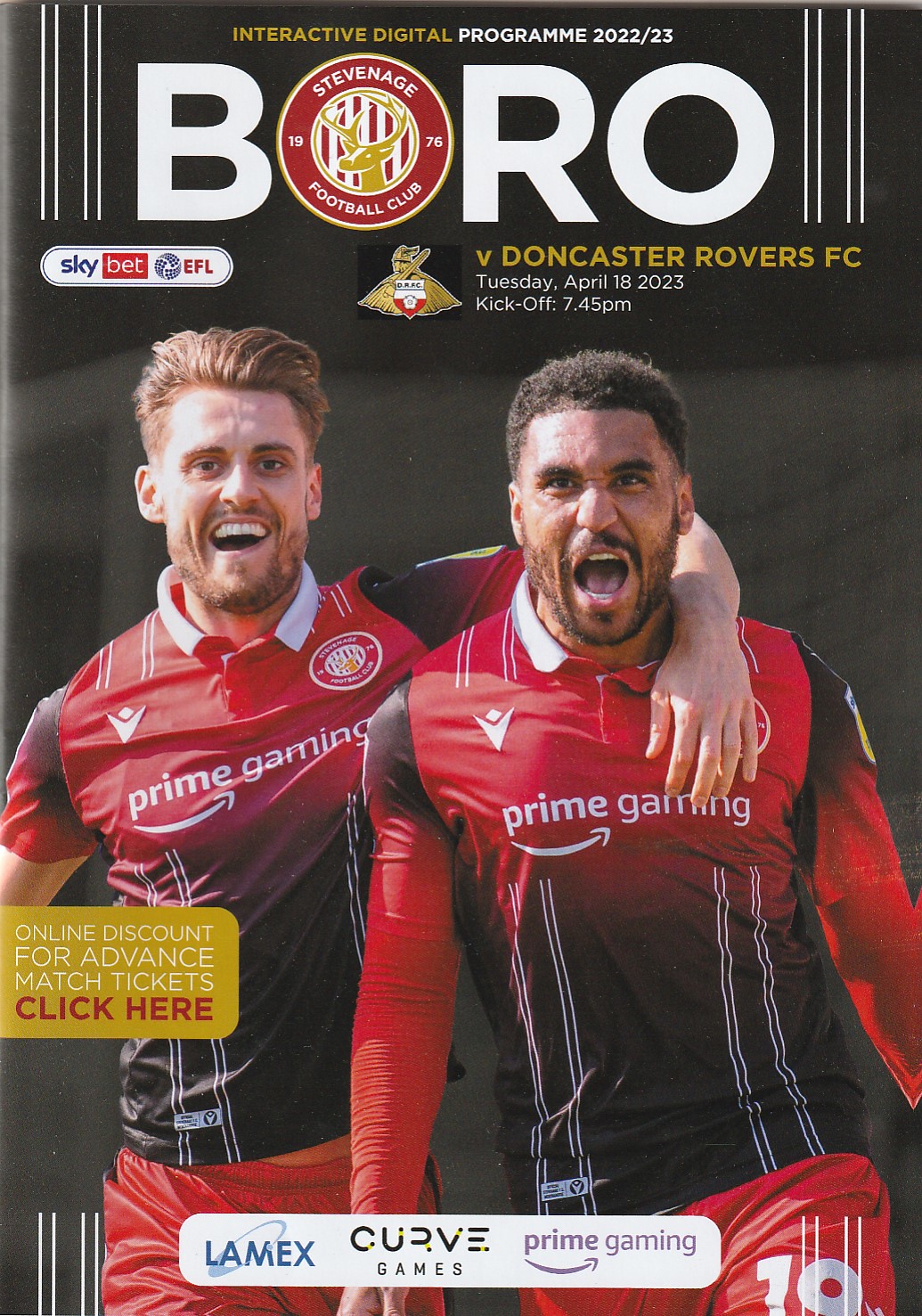The cover of this interactive digital program for the 2022-23 season features a vertically aligned rectangular image with a black and gray background, representing stadium stands. The top prominently displays the title "BORO" in white uppercase letters, except for the first O, which is decorated with a red background and a deer symbol in the center, further outlined in gold, and labeled "Stevenage Football Club". Above this, in gold letters, it reads "Interactive Digital," followed by "Program 2022-23" in white.

Beneath the title, the image announces the match details in gold and white text: "V. Doncaster Rovers FC," "Tuesday, April 18, 2023," and "Kickoff 7.45pm." The center of the image prominently features two soccer players, shown in mid-cheer with wide, open-mouthed smiles. The player on the left, with combed-back short brown hair and matching facial hair, has his arm around his teammate. On the right, the player, who has short black hair and a scruffy beard, is also gleefully shouting. Both players are sporting red and black uniforms with "Prime Gaming" and the Amazon arrow logo printed on their shirts.

The rest of the cover includes several sponsor logos at the bottom: Lamex, Curve Games, and Prime Gaming. Additionally, a small oval in yellow on the left advertises an "online discount for advanced match tickets" with a "Click here" prompt. The overall design emphasizes the excitement and spirit of the upcoming match between Stevenage Football Club and Doncaster Rovers FC.